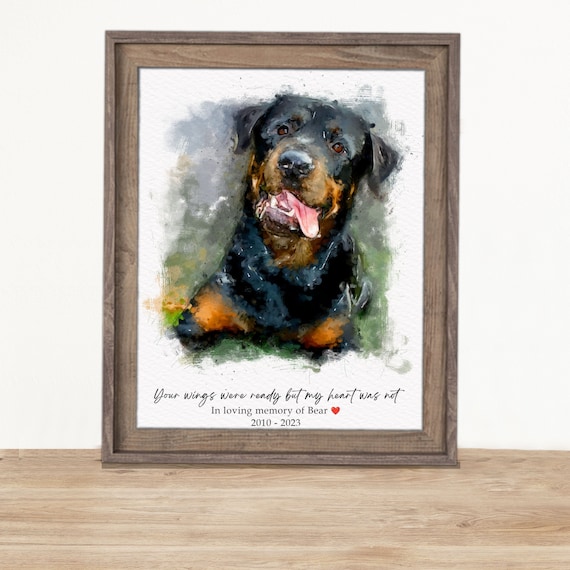This image features a vertically rectangular photograph of a painting, framed in a dark brown wood frame with a white mat. The setting is indoors, with the frame positioned on a light wooden floor and leaning against a white wall. Within the frame, the painting captures a large black dog with a black nose, short black ears, and reddish-brown accents on its face, neck, and legs. The dog's pink tongue is peeking out as it looks directly at the viewer, appearing to be positioned outdoors on grass. Below the dog, the painting bears an inscription in black cursive text: "Your wings were ready, but my heart was not. In loving memory of Bear, 2010-2023," accompanied by a small red heart next to the name Bear. This touching portrait serves as a memorial to a beloved pet dog that has passed away.